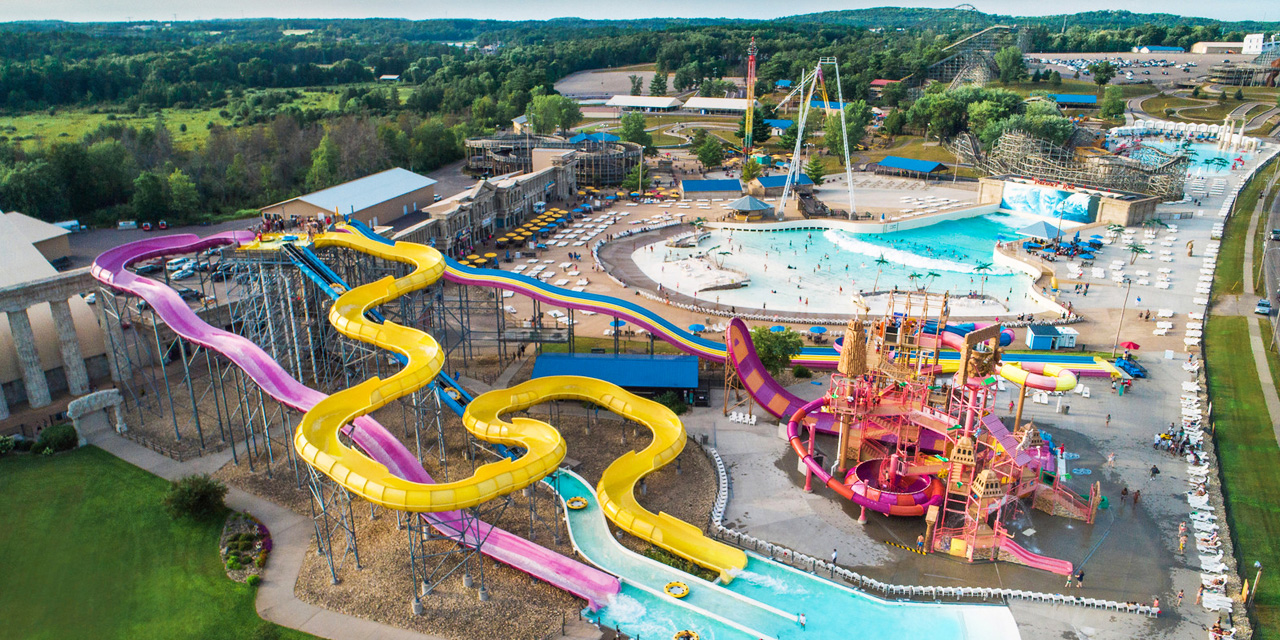This aerial photograph of a bustling water park on a sunny day showcases a vibrant array of attractions aimed at all ages. In the foreground, a series of colorful water slides dominates the scene, featuring a prominent yellow slide with complex twists and turns, accompanied by nearby red, blue, and multicolored slides. Also evident is a large pink and yellow slide, each emptying into their respective pools at the bottom, equipped with inner tubes for riders. Adjacent to these, a more straightforward purple slide runs parallel, contributing to the playful maze of chutes.

Towards the right, a lively children's splash pad is visible, where kids can freely run and get soaked by various water features. Behind this area lies a spacious wave pool, slightly populated with swimmers, surrounded by clusters of white lounge chairs that stretch along the right side of the photograph and behind the pool. The park appears sparsely attended, with visitors scattered sporadically throughout the facilities.

In the backdrop, a few buildings sit amid a picturesque setting, bordered by trees and a small field to the left. The overall scene epitomizes a family-friendly retreat, filled with a diversity of slides and water-based activities against a charming, natural backdrop.